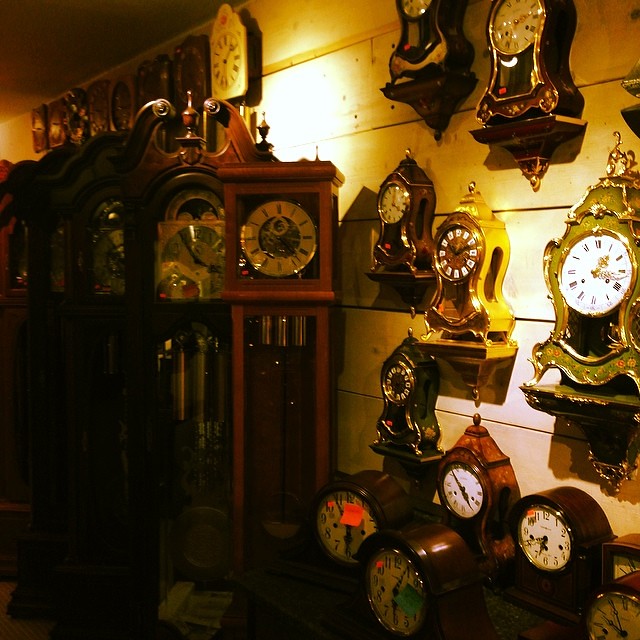This color photograph captures a slightly dimly lit room filled with a variety of ornate, antique-looking clocks displayed in a store setting. The main wall, which has a light brown wooden finish, features shelves holding numerous small clocks of different shapes, sizes, and colors. Some clocks are gold with white faces and black digits, while others are brown wood with white faces. Pink price tags are visible on a few of the clocks. To the left of the image stands a large, tall grandfather clock encased in dark wood with chimes inside its case. Several more grandfather clocks are visible in the background, each flanked above by a row of smaller clocks. The table below the shelves also holds an array of antique clocks, contributing to the room's rich, classic aesthetic. The photograph is devoid of any text, people, animals, buildings, or motorized vehicles, focusing entirely on the intricate collection of clocks.